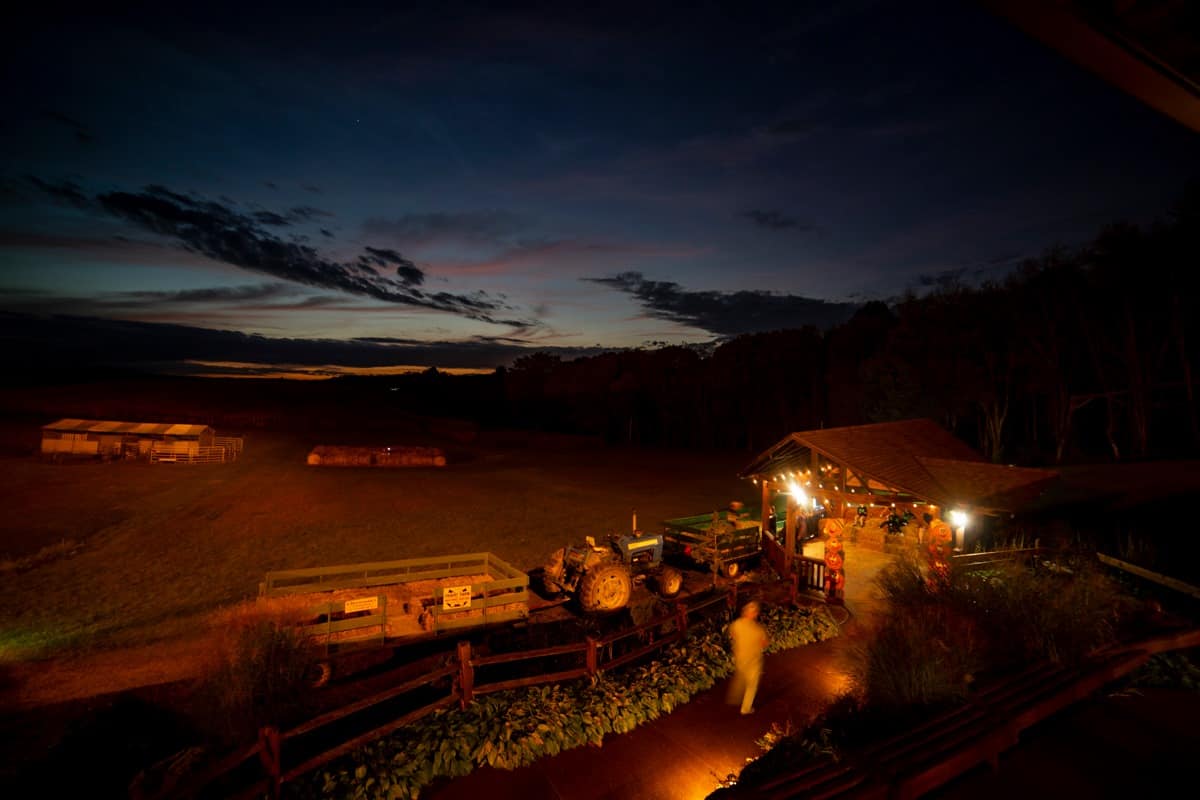This is a detailed nighttime photo taken at a farm, just after sunset. The sky gradates from a lighter blue towards the horizon to a deep, cloud-filled dark blue above, with hints of cream and purple tones breaking through the clouds. In the foreground on the right, a rugged, one-story building with white and gray panels and a wooden fence encircles it, lit with white string lights along the edge of its brown roof. Inside, bales of hay are stacked and people are sitting on them, suggesting a social gathering. A walkway lined with green plants and bushes leads up to this building, with a blurred person walking towards it.

To the left foreground, a tractor with very large wheels is pulling a hay wagon loaded with bales of hay, moving towards the right. In front of the tractor, another wagon is visible. The farm field surrounding this scene shows green growth, probably crops, and is bordered by tree lines on the right. This idyllic, picturesque setting is illuminated softly by scattered lights, enhancing the farm's rugged charm against the twilight sky.